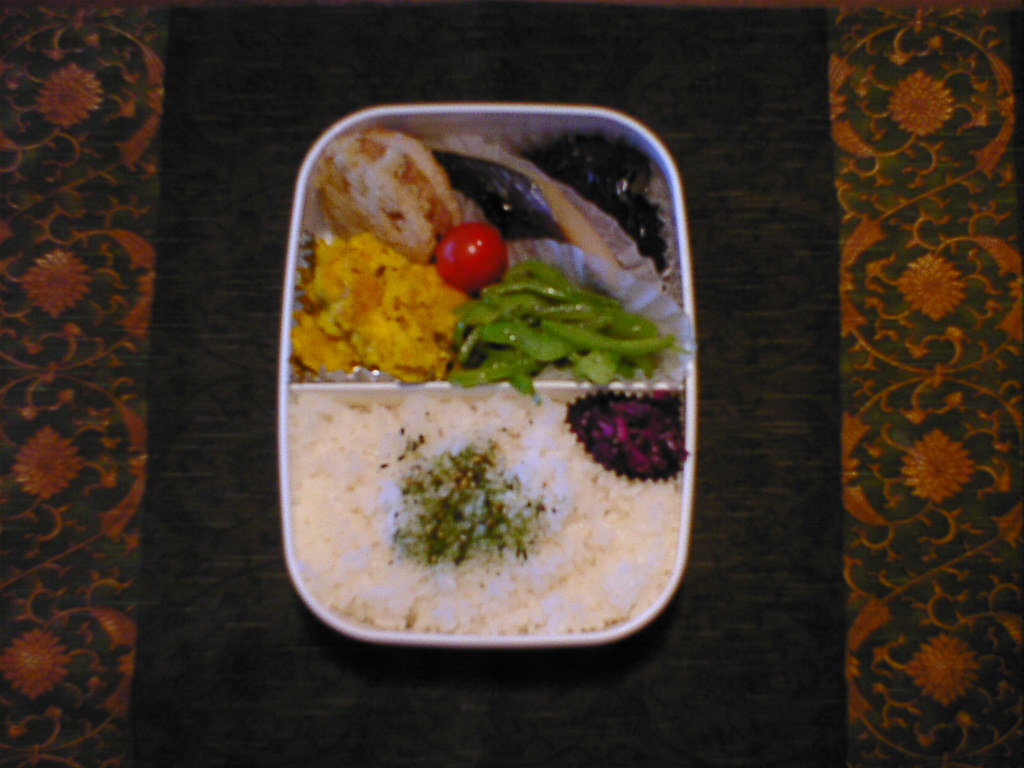The image depicts a meticulously arranged bento box, set against a decorative background featuring red and black borders adorned with intricate chrysanthemum flowers and winding vines. The bento box itself is a silver, aluminum container divided into two compartments. The lower compartment contains a bed of white rice with green seasoning and a small purple item near the top right corner. The upper compartment hosts a variety of foods, including green beans or lima beans, a red circular item resembling a tomato, brown and whitish-brown items similar to scrambled eggs or peppers, and a dark substance in the top right corner. Each section of the bento box's contents is neatly separated, possibly by cupcake papers, highlighting the traditional and aesthetically pleasing presentation typical of Japanese cuisine.